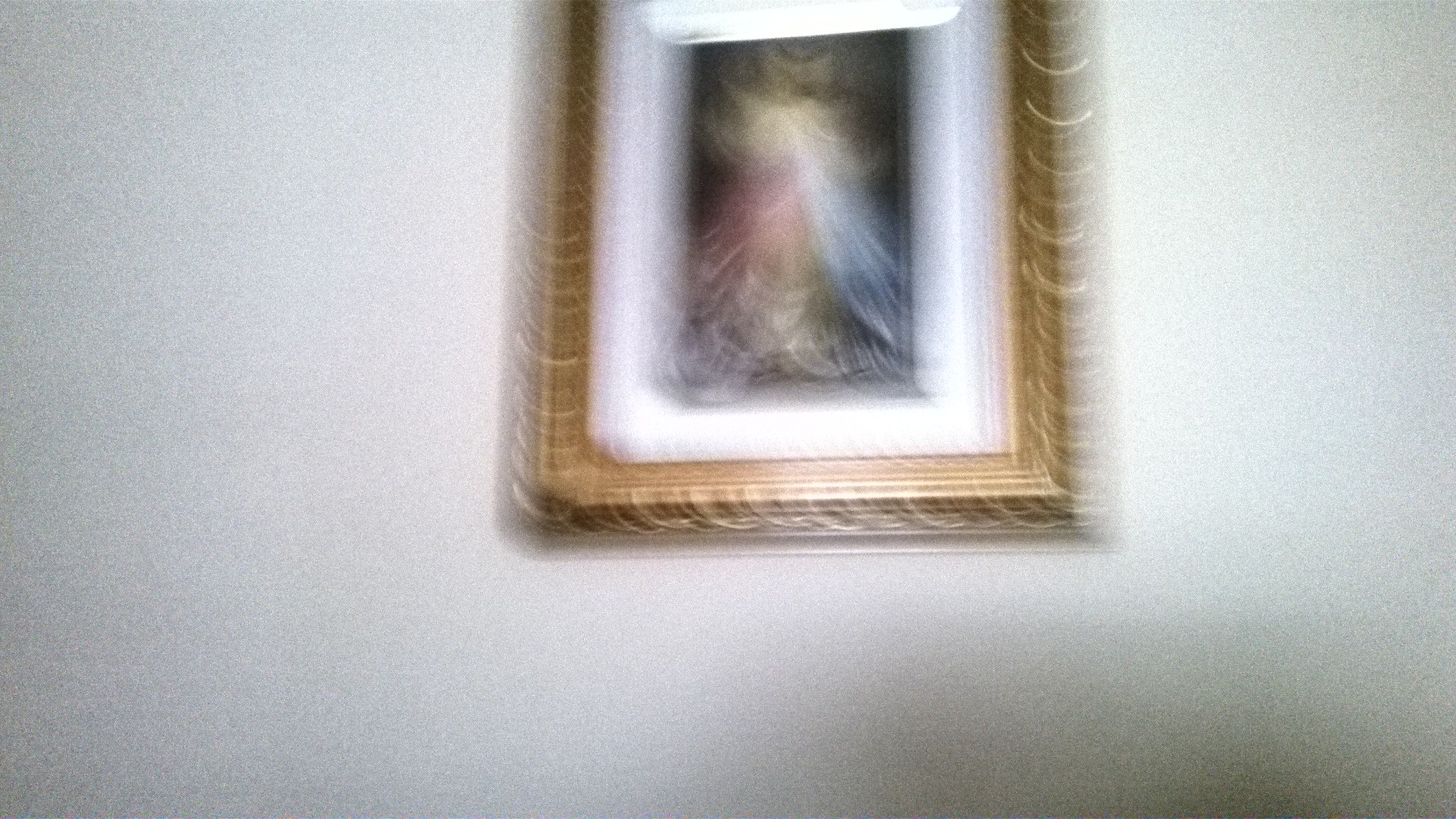The photograph depicts an art piece mounted on a white wall, captured in a blurry manner that makes discerning the details challenging. The art piece is enclosed within an ornate, golden frame, which is hung vertically. The frame features a white mat surrounding the central artwork. The artwork itself has a black background and seems to depict a figure, perhaps a person adorned in a long, draped outfit. The figure appears to have various colors, possibly including yellow, white, red, and blue, though the exact details are obscured due to the photograph's lack of focus. There is also a shadow cast on the wall behind the photographer, hinting at lighting from behind. The photograph offers no additional context about the setting or the specifics of the artwork, leaving its exact nature ambiguous.